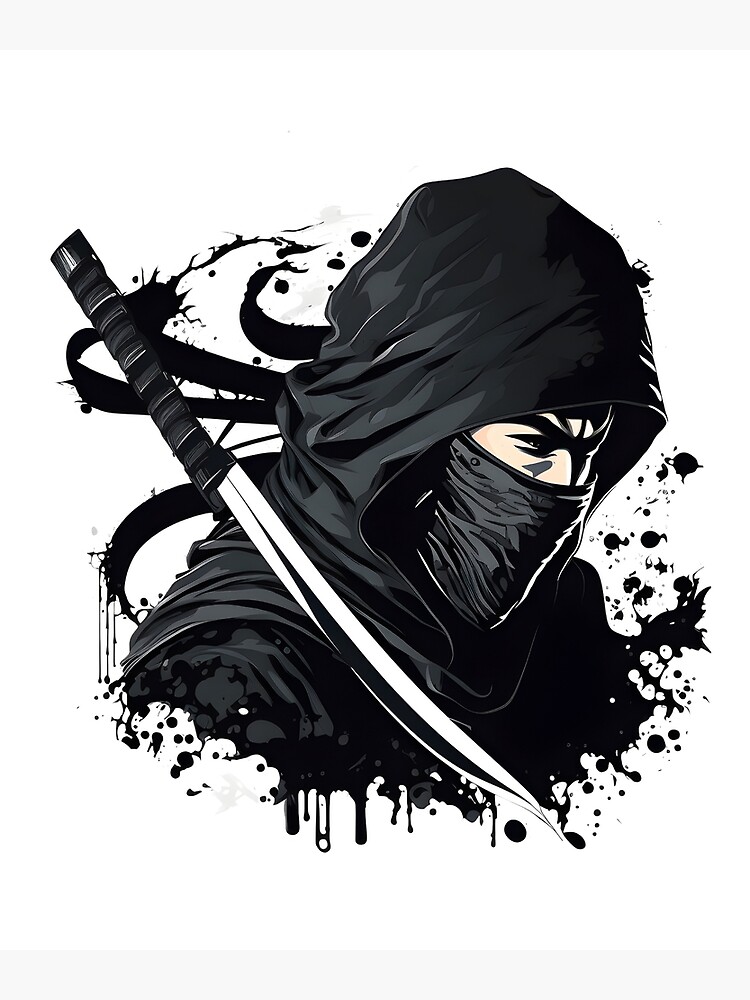A detailed depiction in predominantly black and white, with subtle peach tones, features the upper part of a hyper-focused ninja warrior. The ninja, wearing a black hood and a face mask that covers his nose, has prominently furrowed brows and thick black eyebrows. His eyes, partly closed with intense black pupils, are directed towards the bottom right corner.

The ninja's attire includes a black cowl with pointed ends both upwards and downwards, blending into an intricate pattern of ink splatters and blotches that suggest motion and intensity, with some white specks atop the black blotches. Flowing black straps trail behind him, adding to the dynamic composition.

On his shoulder rests a large ninja sword, its long black handle leading to a slender, silver blade with an extremely fine point, extending downward behind his back. Though the figure is heavily stylized, with ink running along the edges and creating a sense of bleeding into the background, it's likely an AI-generated image, devoid of any descriptive text. The overall visual impact is one of a focused, mean-looking warrior, emerging seamlessly from an abstract ink background.